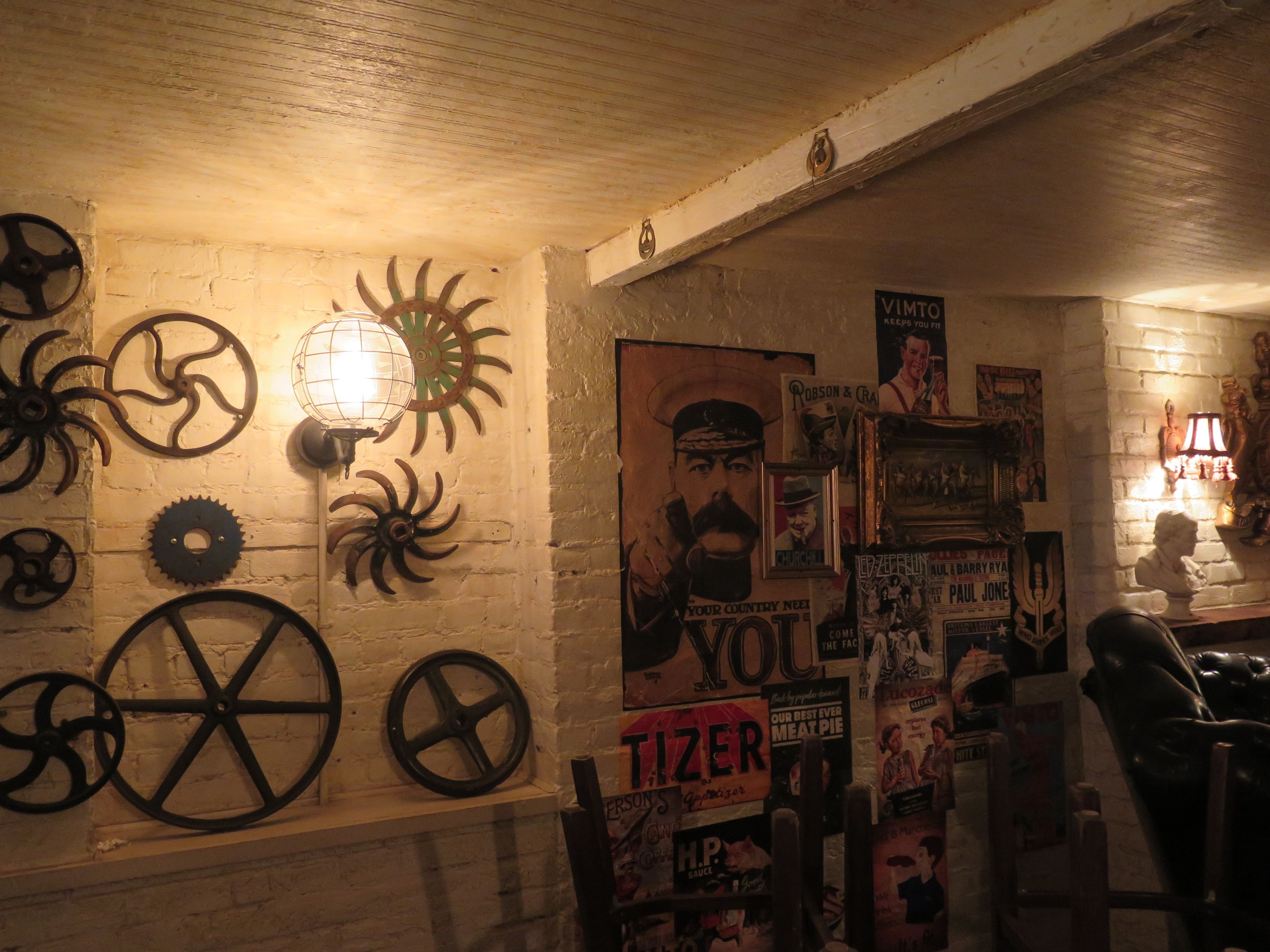This color photo captures an atmospheric basement or underground room with white painted brick walls. The ceiling appears to be made of wood or tile, adding to the rustic ambiance. On the left side of the room, a collection of dark metal gears and wheels in hues of copper, bronze, or burnished brown is prominently displayed. These vary in size and design, with some resembling steering wheels and others like flywheels or suns with radiating spokes.

Illuminating this section is a large, bright, round light hanging near the gear-covered wall. This light resembles a globe or a paper lantern with a checkerboard square holding it up. The middle of the room is adorned with a collage of framed posters, paintings, and political ads. One notable poster features a man with a thick mustache and beard, wearing a navy or army hat, pointing directly at the viewer with the bold message, "Your country needs you" at the bottom. Additionally, a sign reading "TIZER" and another reading "YOU" can be seen among the various images.

The darker part of the room houses a credenza with a bust and a leather chair, adding further character to this intriguing and detailed underground interior.